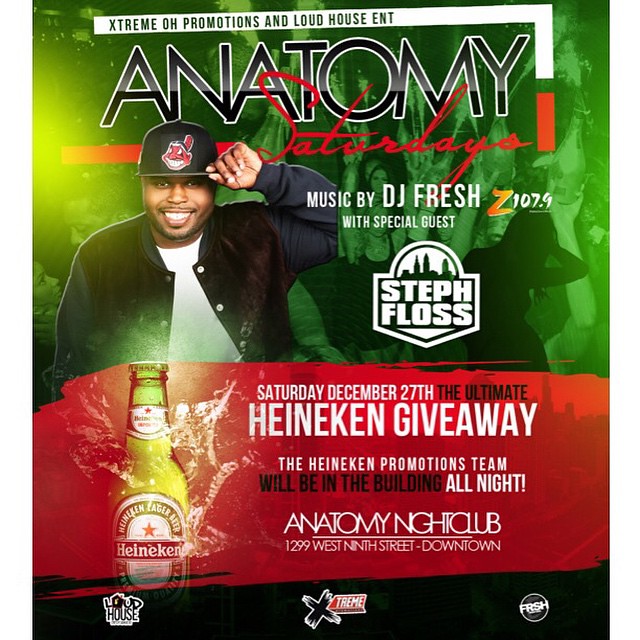The promotional image is a detailed, square advertisement for an event at Anatomy Nightclub. The background reveals a lively club scene with silhouettes of people dancing, bathed in a mixture of green and yellow light that gives a sense of energy and excitement. Overlaid on this backdrop is essential event information presented with distinct typography and design elements. 

At the top, a white rectangular banner features the text, "Extreme O Promotions and Loud House ENT." Below it, in large, bold, black letters outlined in white, the word "ANATOMY" is prominently displayed, with "SATURDAYS" written in elegant red cursive script superimposed over it. 

The central left portion of the image showcases a photo of an African American man with thin facial hair, sporting a black hat emblazoned with an Indian logo. He is smiling and adjusting the brim of his hat. To the right of his photograph, the text in white reads, "MUSIC BY DJ FRESH Z1079" with the "Z" highlighted in orange, followed by, "WITH SPECIAL GUEST STEPHEN FLOSS."

At the bottom of the image, a dynamic red paintbrush-like section stretches across, adding vibrancy to the design. On the left side of this red band is a photograph of a Heineken bottle with splashes of water around it, emphasizing freshness. Adjacent to the bottle, the text announces, "SATURDAY, DECEMBER 27, THE ULTIMATE HEINEKEN GIVEAWAY. THE HEINEKEN PROMOTIONS TEAM WILL BE IN THE BUILDING ALL NIGHT." It concludes with the location details, "ANATOMY NIGHT CLUB, 1299 WEST 9TH STREET, DOWNTOWN."

This sophisticated design effectively combines photographic realism with graphic design and typography, creating an eye-catching and informative advertisement for the upcoming event.